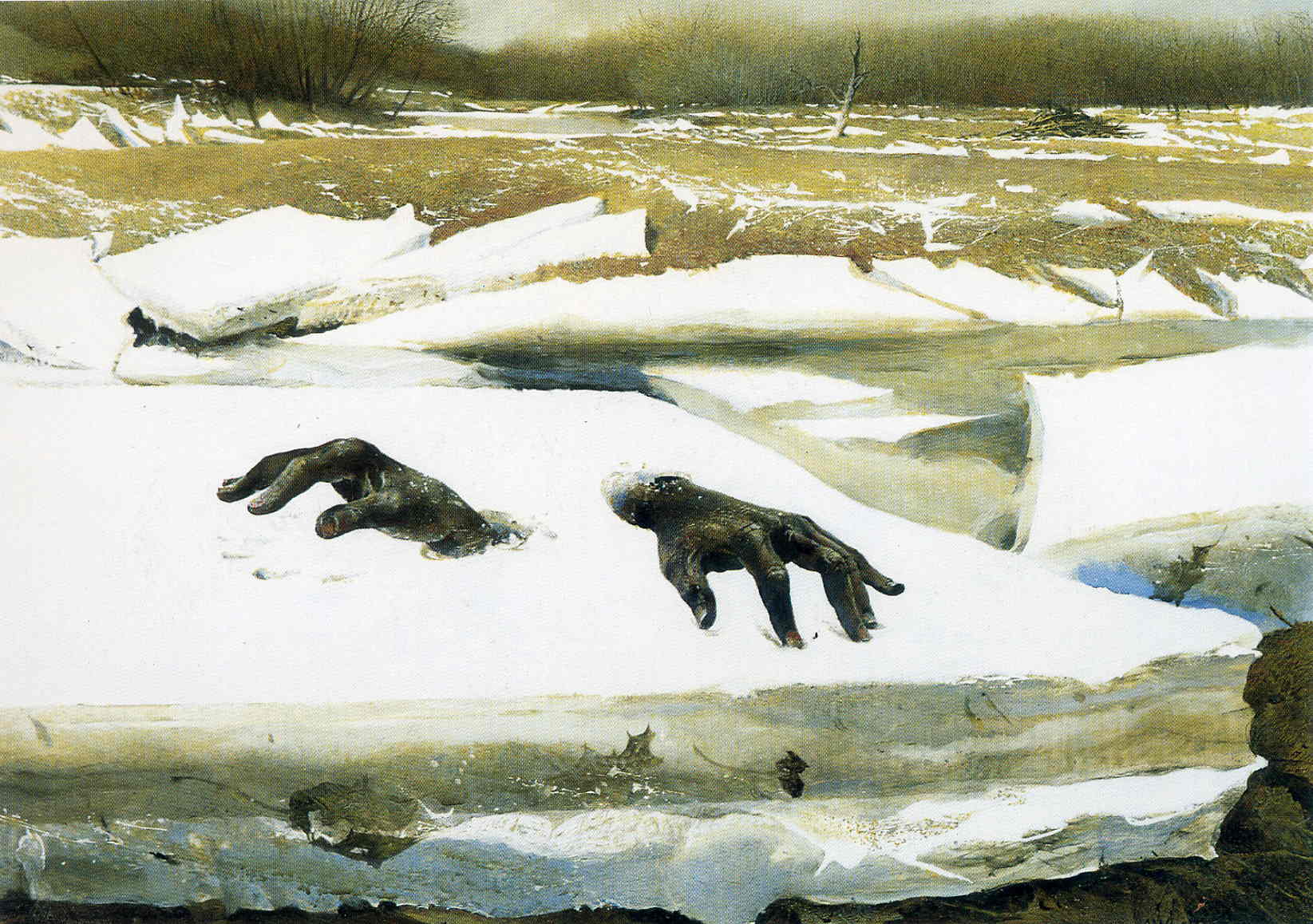This painting, titled "Breakup" by Andrew Wyeth, depicts a haunting outdoor winter scene, rendered with meticulous detail and a slightly ghoulish atmosphere. In the foreground, a pair of black hands emerge dramatically from the top of a large rectangular ice floe, their position suggesting a lifeless, almost ghostly presence. The hands rise through two circular openings in the ice, with the right hand seemingly playing an invisible piano and the left hand lifted slightly into the air.

The ice floe itself is predominantly white at the top, transitioning into shades of gray and green along its cut side. Surrounding the main ice floe are various smaller chunks of white ice, floating in a brownish-green expanse of water that appears to flow towards the viewer. The water hints at a thaw, juxtaposing the solid ice and liquid state, enhancing the scene's eerie mood.

In the background, a dense array of leafless trees stands stark against a strip of gray sky on the horizon, contributing to the painting's somber tone. On the left side, patches of green mixed with snow and what appear to be blocks of wood covered in snow add texture and depth. To the right of the emerging hands, a small blue patch suggests water, and in the lower right corner, rocks are piled up, adding to the scene’s rugged and desolate feel. Overall, the painting beautifully captures a moment of unsettling stillness, combining natural elements with an eerie, surreal touch.